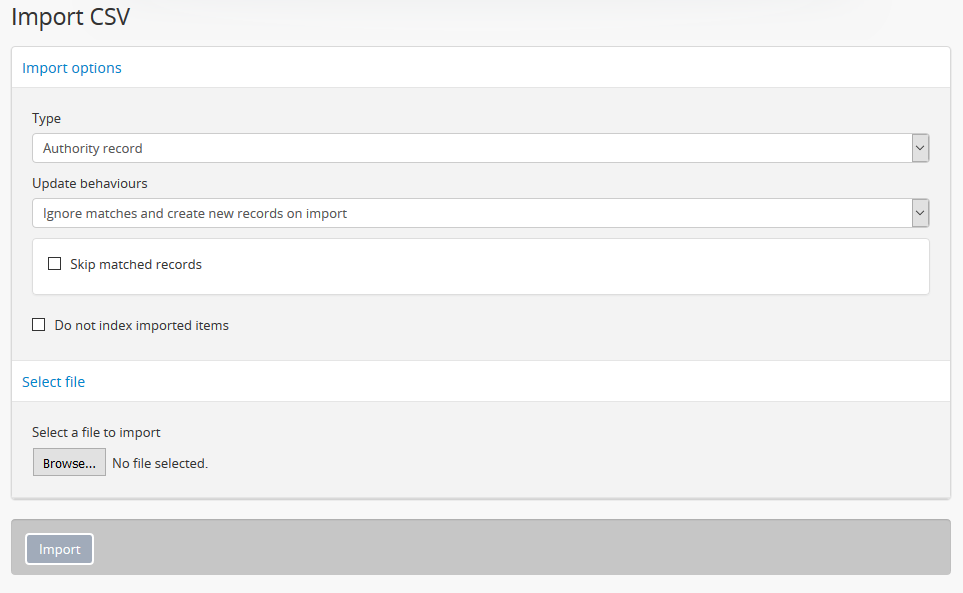This image is a cropped screenshot from an unidentified website or software application, showcasing a form-style section specifically for importing CSV files. The section is titled "Import CSV." Below the title, there is a grey-background window presenting several import options.

The first option is a drop-down menu labeled "Type," with "Authority Record" currently selected. Next, there is a drop-down menu labeled "Update Behaviours," which shows the selected option as "Ignore Matches and Create New Record on Import." Further below, there are two checkboxes: one labeled "Skip Matched Records" and another labeled "Do Not Index Imported Items." Neither checkbox is selected.

The second major section of the form is "Select File," featuring a grey "Browse" button intended to open a file explorer for file selection. No file has been chosen yet. At the bottom, there is a dark grey "Import" button that presumably initiates the CSV import process once all options have been configured and a file has been selected.